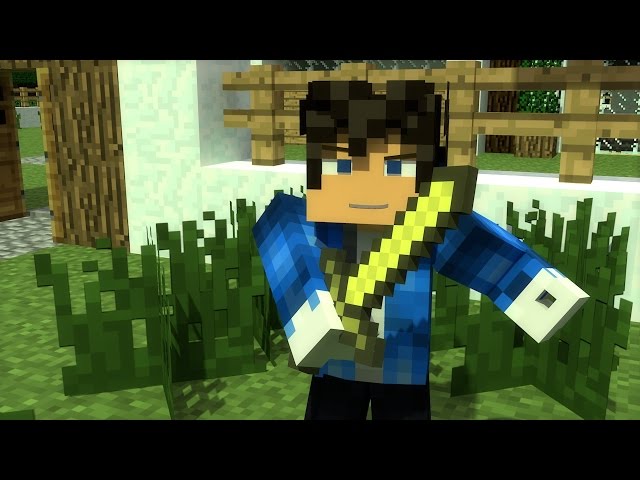The image depicts a heavily pixelated, computer-animated character reminiscent of Minecraft. The figure features a simplistic block design, including a rectangular block head, long rectangular arms, black hair, and blue eyes. They wear black pants and a blue shirt with white sleeves and a white button-down front, though no buttons are visible. The character appears to be holding a green and olive-colored sword across their body, despite the absence of visible hands. Behind the character is a brown wooden fence and lush, green, animated-style grass. To the left, there is a brown doorway with more grass beside it. The overall low-resolution quality evokes a nostalgic feel akin to early 1980s computer games.